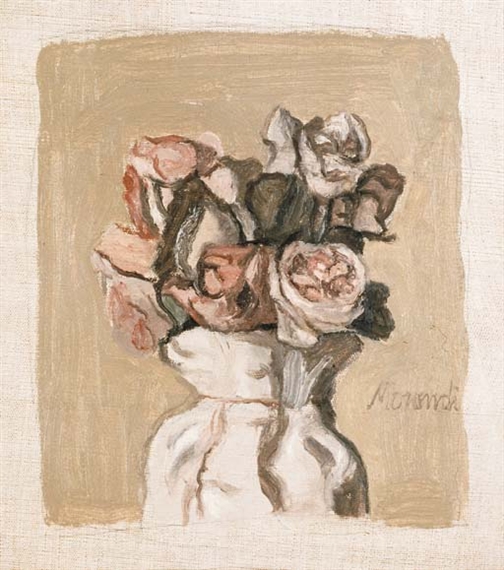The painting depicts a bouquet of flowers, possibly roses, with blooms in shades of pink, white, and red, and accompanied by brown and green leaves. The bouquet appears to be placed in a vase draped with white fabric, tied near the top with a string or rope. The background is a medium to dark brown with a lighter brown or beige border framing the composition. Featured prominently in the painting is the artist's name, which seems to be "MORSIND" or similar, rendered in text. The overall style of the painting is simple and possibly watercolor, not striving for realism but clearly illustrating the subject matter. The use of varied browns, along with occasional orangish-pink tones, contributes to a subdued but harmonious color scheme.